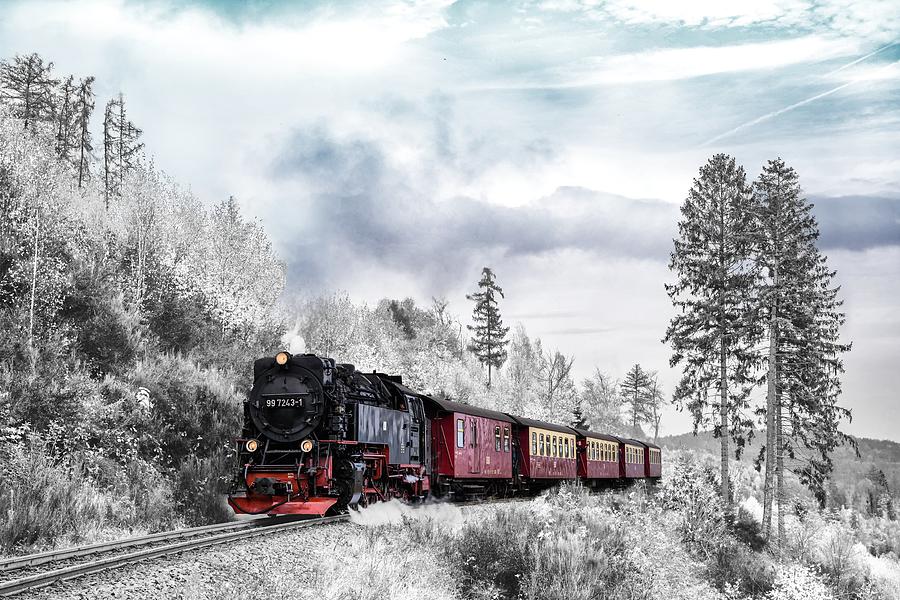The photograph captures a wintery mountainous landscape on an overcast day. The square frame predominantly features a cloudy sky, with grey and white clouds filling the upper portion. The scene shows a snow-covered terrain with a variety of trees; scraggly pines, hardwoods, and scrub brush, all lightly powdered with snow. The focal point is a black steam engine train, distinguished by its red cow catcher and the number 997243-1 prominently displayed on its front. The engine is pulling five red cars; the first is a caboose-like car, while the remaining four passenger cars each have yellow frames around their windows. The train, emitting smoke from beneath, travels along tracks that weave through the snowy, tree-laden hills on either side.